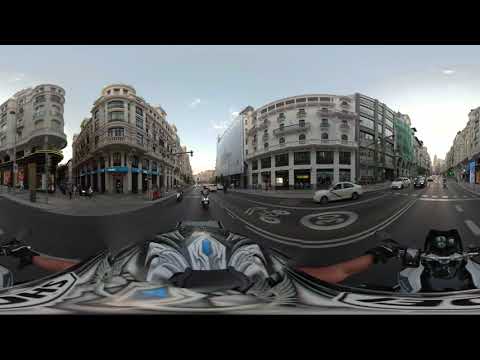The image reveals a city street captured from the vantage point of a motorcycle helmet, suggesting the use of a 360-degree camera. The angle displays two intersecting streets, characterized by dark gray concrete with white road markings and a bicycle lane. The view appears slightly off-center, revealing multiple gray, multi-story buildings, approximately two to four stories tall, possessing an old-world charm with visible columns, faded paint, classical windows, and balconies. Some buildings show signs of wear, enhancing their historical appearance. There's a horizontal black stripe framing the top and bottom of the image.

In the warped, panoramic view, the white motorcycle to the right features prominently with the rider's hands gripping the handlebars, one appearing on the far right and the other improbably on the left side of the frame due to the image's distortion. The rider's helmet, with a gray and white design, is also visible, adding to the dynamic composition. The sky is a light blue, accented with a few white clouds, adding a touch of serenity to the urban scene. Notable details include a green scaffolding on one of the buildings to the left, a large billboard on another building front, and light oncoming motorcycle traffic, hinting at a European, possibly German, setting.